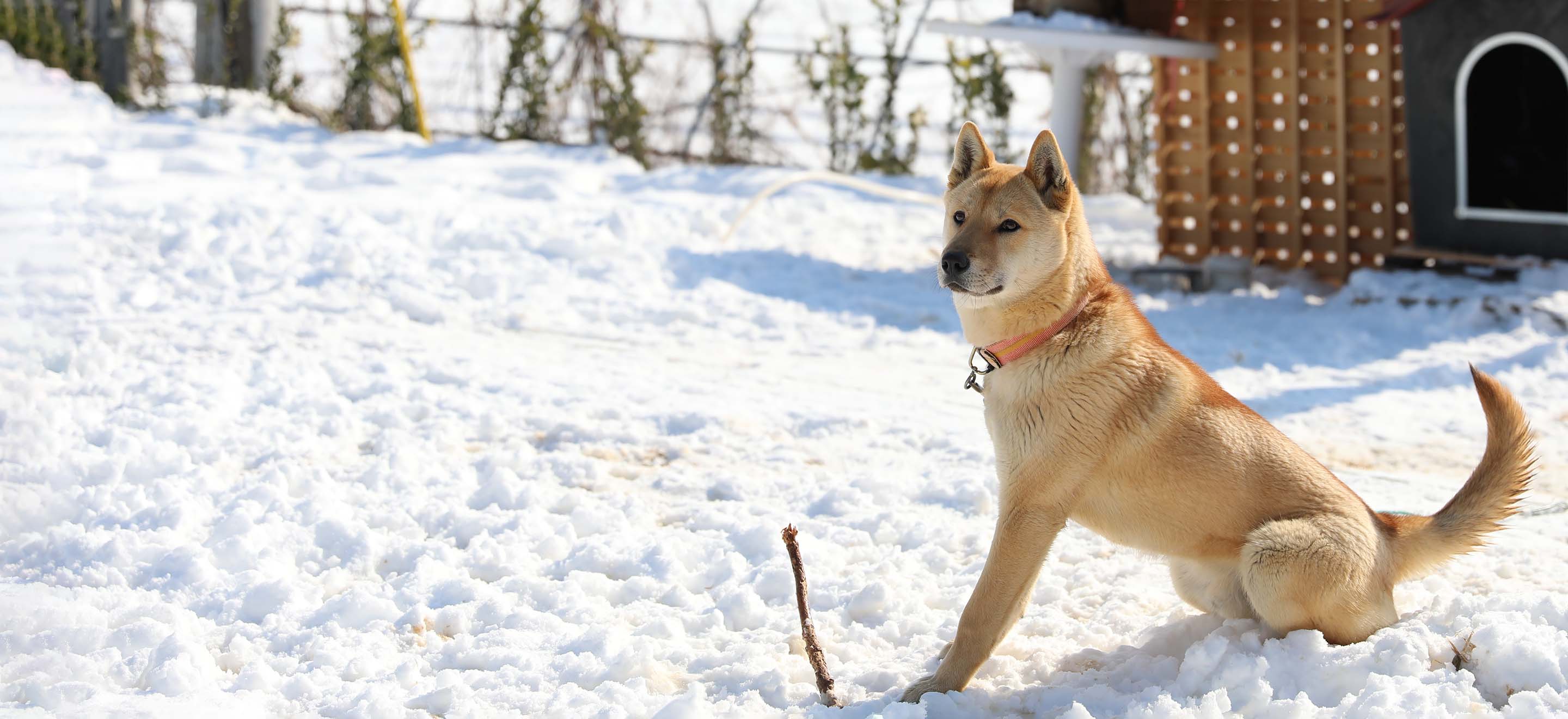In this outdoor image, we see a snowy yard dominated by a muscular, large blonde dog with pointed ears standing upright. The dog, a light tan to golden brown color with lighter cheeks, sports an orange collar with a central metal piece. It stands with its body facing left but its head turned slightly towards the viewer, curiously eyeing something in the distance. The dog's long tail is raised and curves gently to the left, and its black nose stands out against its lighter fur. The dog appears to be playing with a stick partially protruding from the snow to its left.

In the background, there is a thin wire fence adorned with vegetation running diagonally from the top left to approximately three-fourths of the way to the top right. Nestled in the upper right corner is a doghouse with dark gray walls, white trim around its black, rounded entryway, and a wooden grate with holes on one side. The sunny day highlights the thick, expansive snow that blankets the yard, positioning the dog as the central focus of this tranquil, wintry scene.